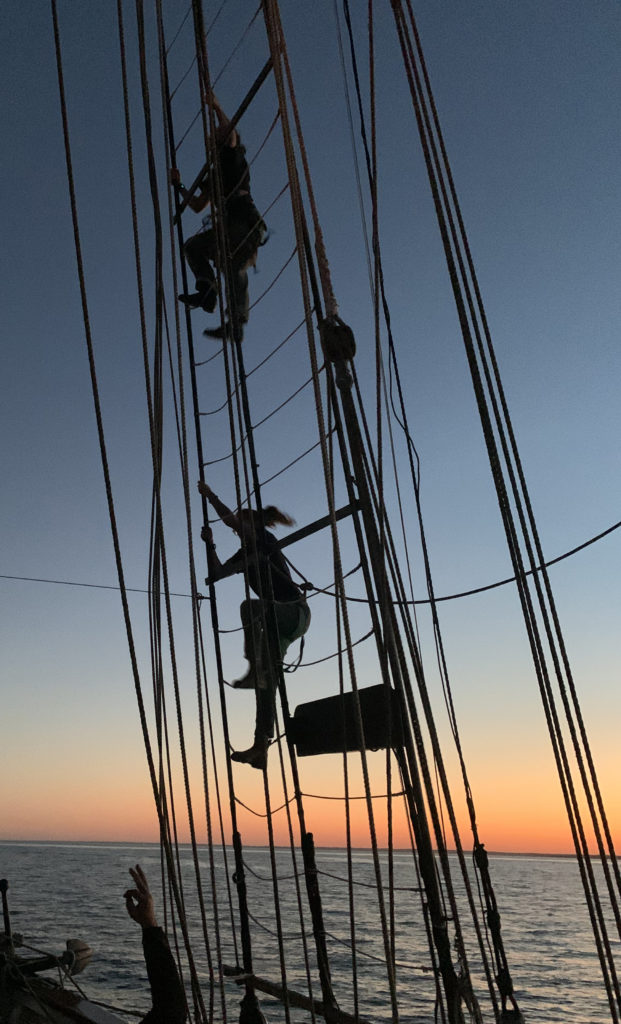The photograph captures a serene maritime scene at either sunrise or sunset, characterized by a gradient sky transitioning from dark blue at the top to bright orange and yellow near the horizon. The sea, depicted as fairly calm with small waves, stretches out in the background. Central to the image is the silhouetted mast of a sailboat adorned with rigging and cables, resembling a complex rope ladder. Two figures, whose features are obscured by shadows, are seen climbing the mast, seemingly secured by safety ropes. The climbers might be engaged in some form of maintenance or repair at the top, which is not visible in the frame. In the foreground, a man's hand is prominently shown making an OK gesture towards the climbers, suggesting supervision or communication, though the rest of the person is not visible. The image, oriented in a landscape format, creates a captivating blend of human activity and natural beauty.